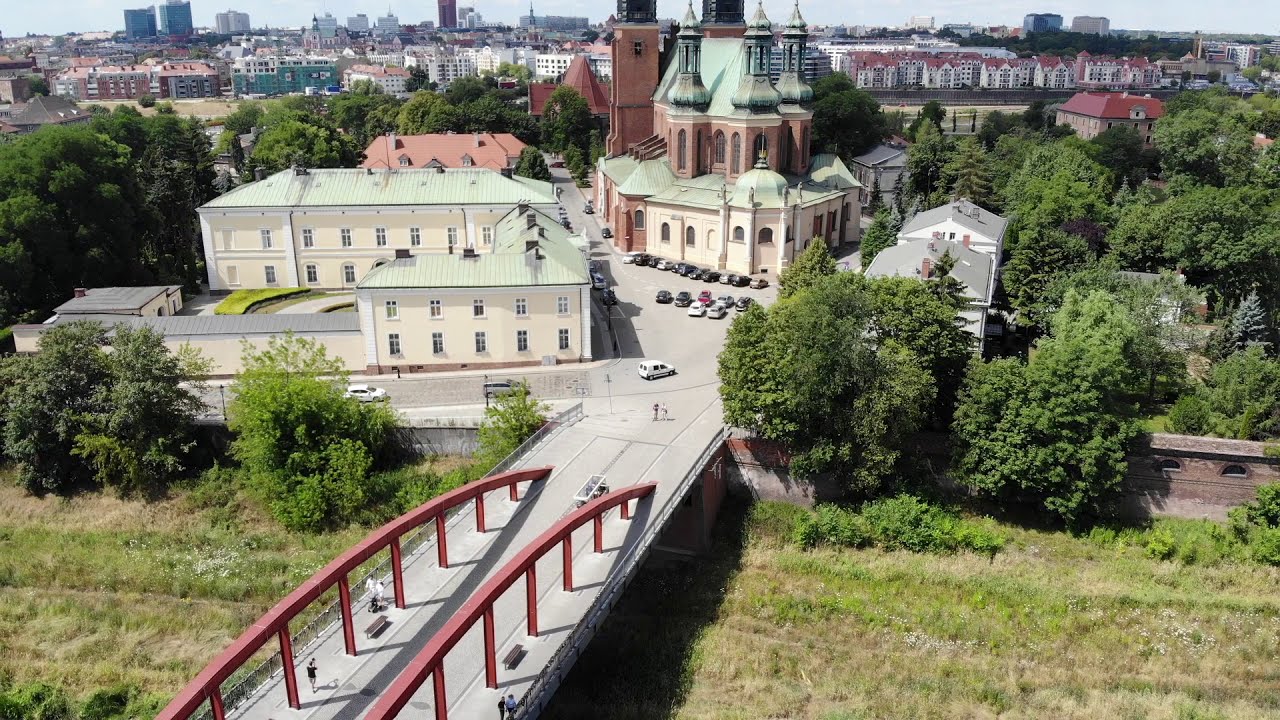This horizontal, rectangular aerial image, likely captured by a drone, showcases a densely populated European city, possibly Eastern European, centered around a prominent set of buildings resembling a church or castle. The main focal point is an elaborate church-like structure with at least three steeples, some of which are so tall they extend beyond the top edge of the image. This grand building, constructed from yellow brick with a green roof, is flanked by small and large adjoining structures, possibly indicating a complex that includes a school or other related facilities. 

In the foreground stretches a pedestrian bridge with red railings traversing a grassy area and leading to steps that descend to the pavement surrounding the central buildings. The bridge, which also accommodates foot traffic on a road, complements the scene with patches of greenery and several parked cars in front of the main edifices. Encircling this area are lush green trees, contributing to a park-like ambiance amidst the urban environment.

In the distant background, a dense cityscape with numerous buildings, including skyscrapers, extends towards the horizon, creating a vivid contrast between the historic charm of the central structure and the modern urban skyline. The horizon itself suggests proximity to a water body, further enhancing the scenic attributes of this European urban setting.